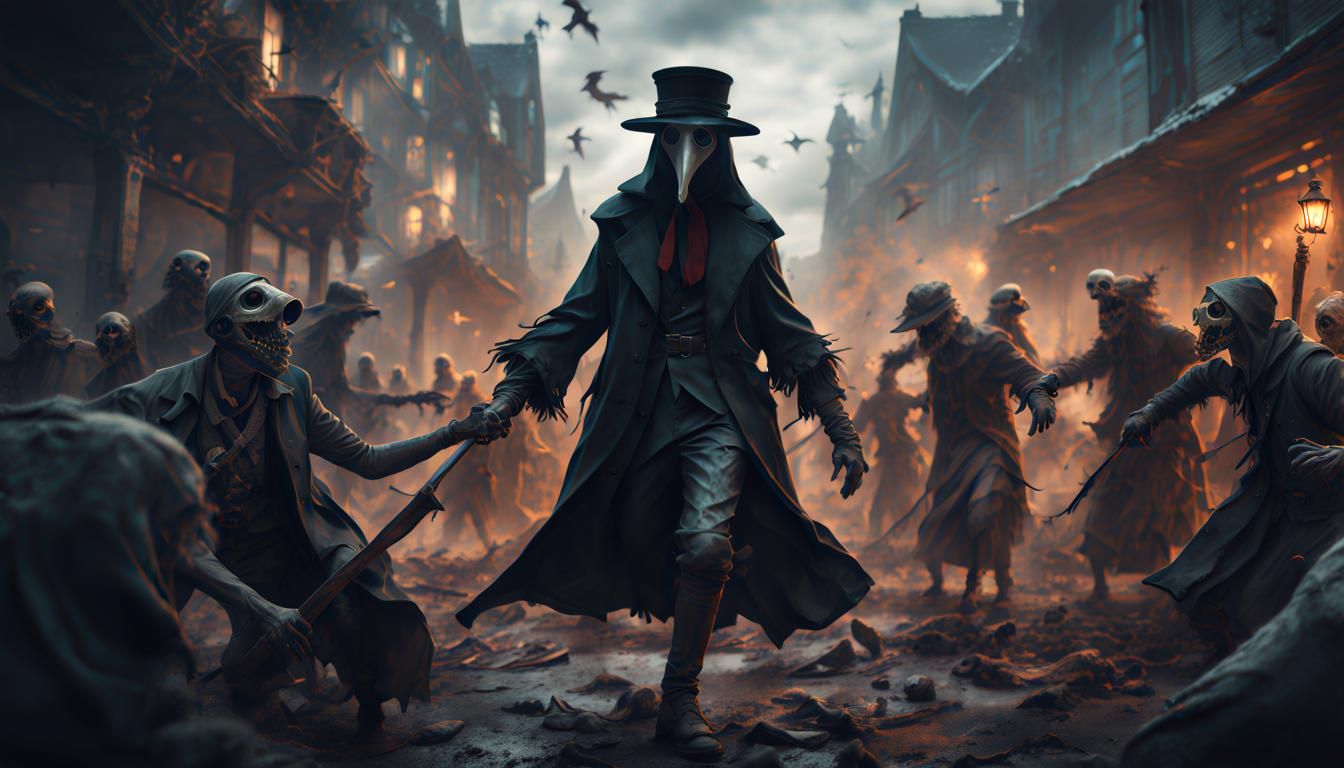The image is a highly detailed digital illustration, possibly AI-generated, featuring a man dressed in a plague doctor costume. He stands at the center, donning a long black overcoat, knee-high leather boots, and a tall black hat with a cape. His face is obscured by a white beaked mask reminiscent of those worn by medieval physicians, and he sports a dark red tie. Surrounding him are skeletal beings with animalistic skulls, clad in long, tattered black clothes, creating an eerie, deathly atmosphere. The setting appears to be a desolate, old-fashioned cityscape, with run-down, dirty buildings reminiscent of an 1800s English town, evoking a Sweeney Todd vibe. The background teems with bats and crows flying amidst the chaos, further enhancing the grim, Halloween-like essence of the scene. The color palette is dominated by somber tones of black, gray, and brown, emphasizing the illustration’s dark and foreboding theme.